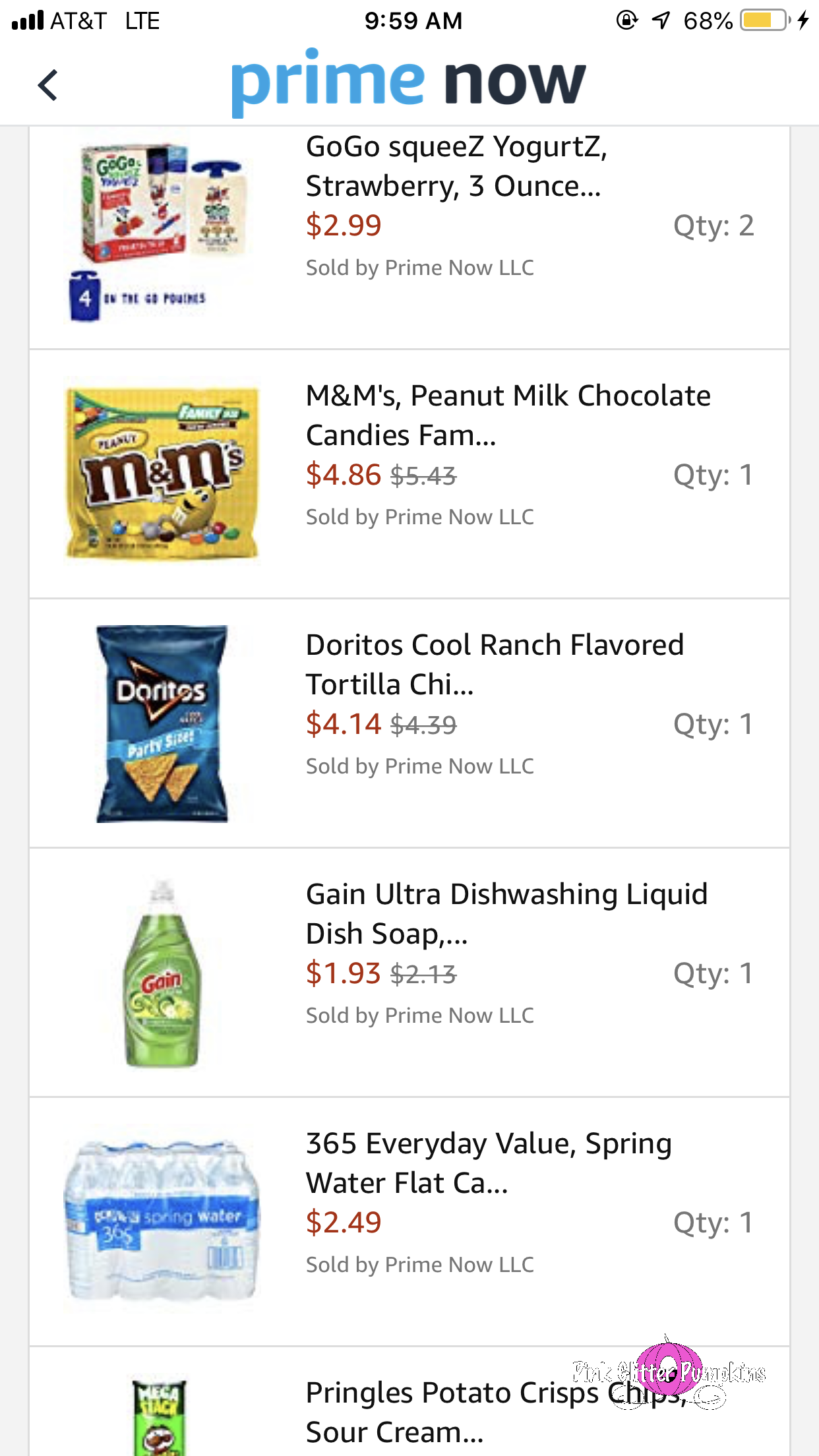The image depicts a smartphone screen displaying the Amazon Prime Now website. At the top of the screen, the status bar indicates that the device is connected to the AT&T network with a full cell signal and LTE data connectivity. It's 9:59 AM, according to the black-font time display, and the battery level is at 68%, shown in yellow, with an icon indicating that it's currently charging. The screen orientation is locked in landscape mode, as denoted by the lock screen icon next to a map icon.

Below the status bar, the Prime Now logo is prominently featured, followed by a detailed list of the customer’s recent orders. The orders include:

1. **Go Go Squeeze Yogurt** - Priced at $2.99 each, with two units ordered.
2. **M&M's Peanut Butter Milk Chocolate** - On sale for $4.86, with one unit ordered.
3. **Doritos Cool Ranch Party Size Bag** - Priced at $4.14, with one unit ordered.
4. **Gain Ultra Dishwashing Liquid Dish Soap** - On sale for $1.93, with one unit ordered. The sale price is highlighted in red.
5. **365 Everyday Value Spring Water** - On sale for $2.49, with one unit ordered.
6. **Pringles Chips** - The image of this item is partially visible, cut off right under the iconic Pringles mascot's face.

Each product is accompanied by an image and a "Sold by Prime Now LLC" label. The Pringles image is particularly noted for being partially cut off, obscuring a portion of the product details.